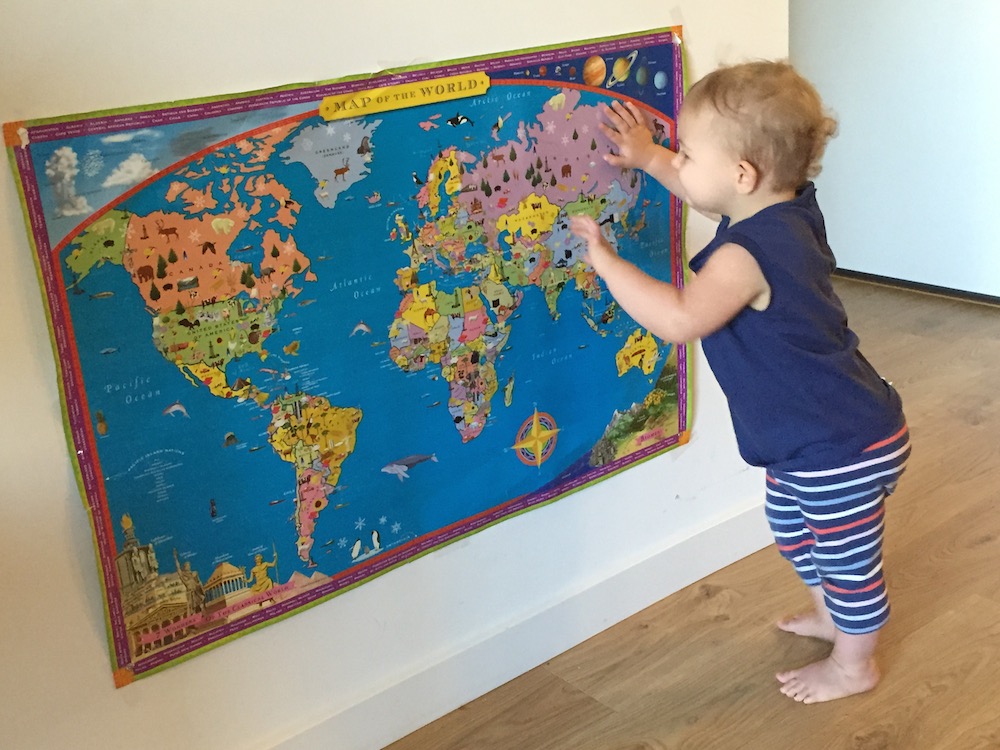In a cozy indoor setting with light brown wooden floors, a joyful baby with short brown hair and a sleeveless dark blue top stands on bare feet, enthusiastically interacting with a colorful world map titled "Map of the World" on a light yellow wall. Positioned on the right side of the image, the baby faces the map on the left, his left profile visible as he touches it with both hands – one on the area of China and the other extending towards the rest of the map. The baby is dressed in vibrant striped pants featuring orange, blue, and white colors, and his radiant smile infuses the scene with a sense of curiosity and wonder. The detailed map is mounted at a height that allows the child easy access, adding to the engaging and inviting atmosphere of the home.